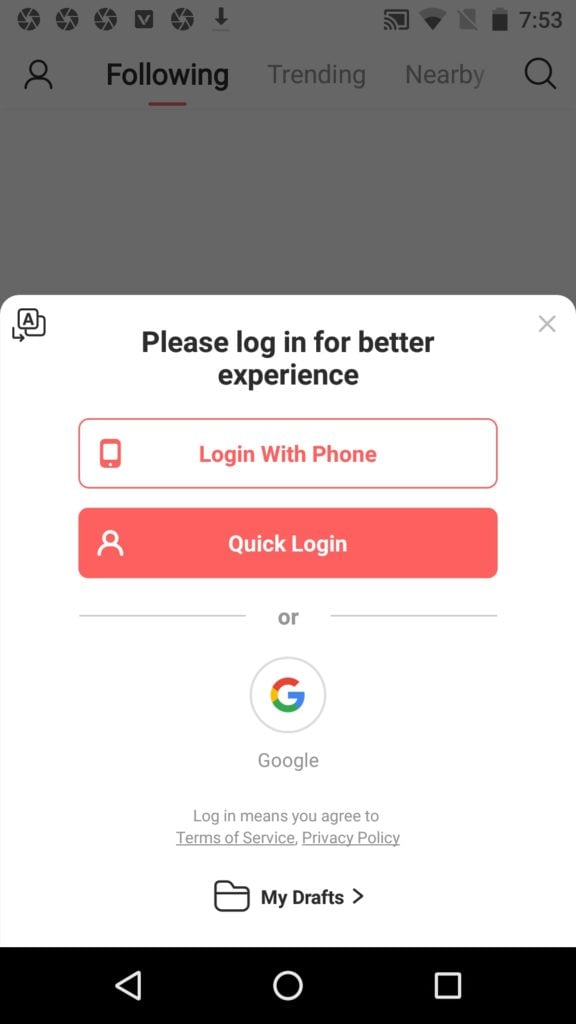The image is a screenshot of a smartphone display. In the top left corner, there is a number "3," while on the top right, there is a "53" accompanied by the text "Texas is following, trending nearby in gray font. Below it, there's a notification icon. The middle section of the screenshot has a message prompting the user to "log in for a better experience" within a red-bordered star icon. The screenshot also features a "Log in with phone" button and a rectangular "Quick login with Google" option, indicating user login options, along with a disclaimer that using these options means agreeing to the "Terms of Service" and "Privacy Policy." There is a black bar at the bottom of the image, and within this bar, on the left side, there are circular and square icons. Various text elements are visible throughout the image, reflecting a typical user's interface on a smartphone.